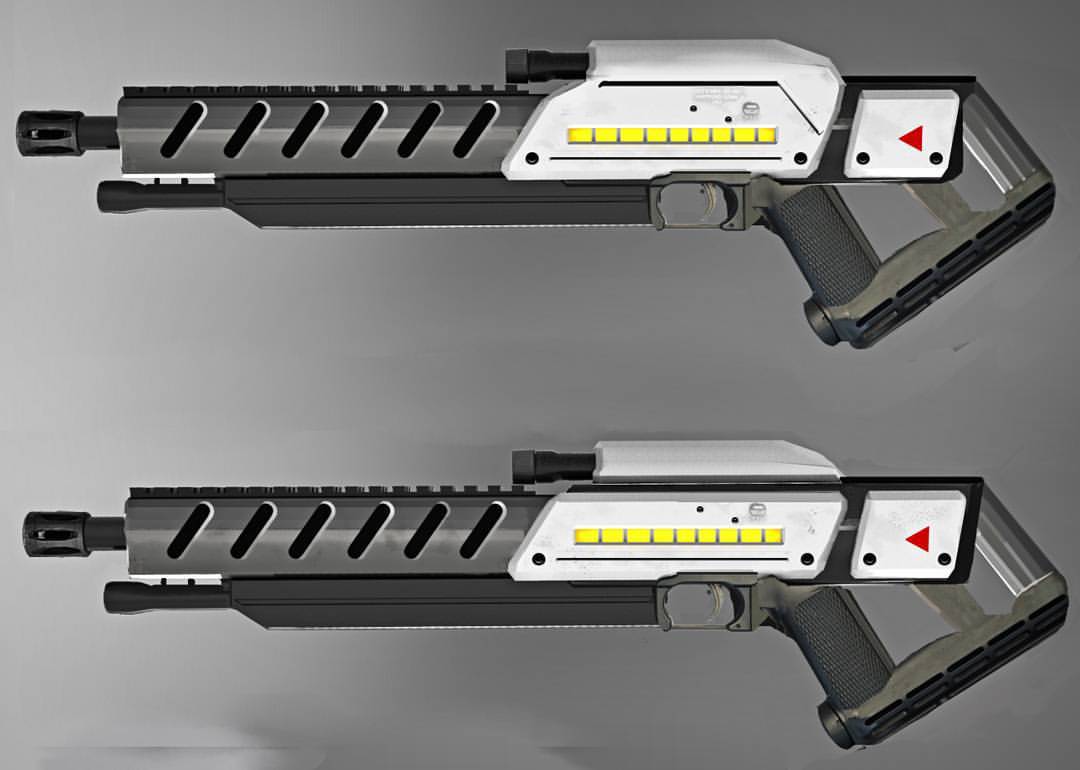The image features two identical, futuristic guns placed one above the other against a gradient grey background. Both guns are predominantly a dark charcoal grey with a slightly narrower barrel that extends outwards and features six diagonal cutout marks. The middle section of each gun is white and adorned with a line of yellow squares, resembling a digital screen. Towards the rear, there is another white section with a red triangle. Each gun is equipped with a scope and an angled handle located behind the trigger, which is enclosed within a standard rectangular trigger guard. The overall appearance suggests a blend between a shotgun and an assault rifle, marked by its sleek, modern design.